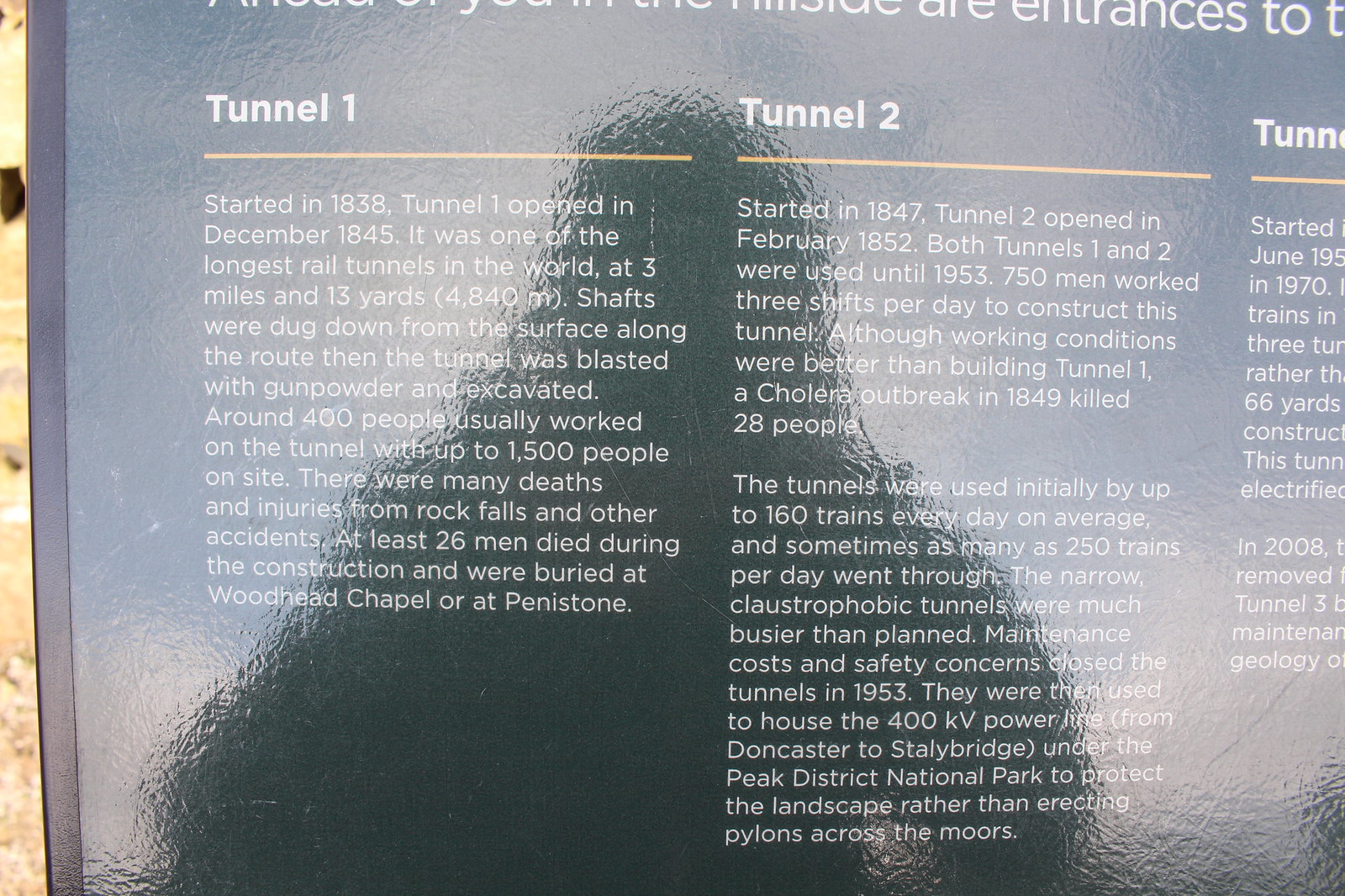This is a color, close-up outdoor daylight photograph of a sign or display describing various historical rail tunnels. The sign, placed outside and likely in a park area, features detailed information in white text with gold lines separating the sections. The reflective black surface of the sign also captures the shadow of the photographer, indicating its glossy finish.

The text describes "Tunnel 1," marked with a gold line under its title. "Tunnel 1" began in 1838 and opened in December 1845. At three miles and 13 yards (4,840 meters), it was one of the longest rail tunnels in the world at its time. Construction involved blasting with gunpowder and excavation via shafts dug from the surface. Approximately 400 people worked on the tunnel, escalating to up to 1,500 people on-site. The construction environment was perilous, resulting in numerous injuries from rock falls and accidents, and at least 26 men died. They were buried at Woodhead Chapel or Penistone.

Additionally, the sign mentions "Tunnel 2," which started in 1847 and opened in February 1852. This tunnel construction engaged 750 men working in three shifts per day in notably better conditions than those of "Tunnel 1." A cholera outbreak in 1849, however, claimed 28 lives. Both tunnels accommodated up to 160 trains per day on average, reaching peaks of 250. Severe maintenance costs and safety concerns led to their closure in 1953. Post-closure, the tunnels housed high-voltage power lines to preserve the Peak District National Park's landscape.

Though partially obscured, a third column on the sign describes "Tunnel 3," initiated on June 19, 1970. The incomplete text suggests that this tunnel involved modern electrification and sophisticated geological considerations for maintenance. The entire sign eloquently narrates the history, construction techniques, and utilization of these significant rail tunnels.